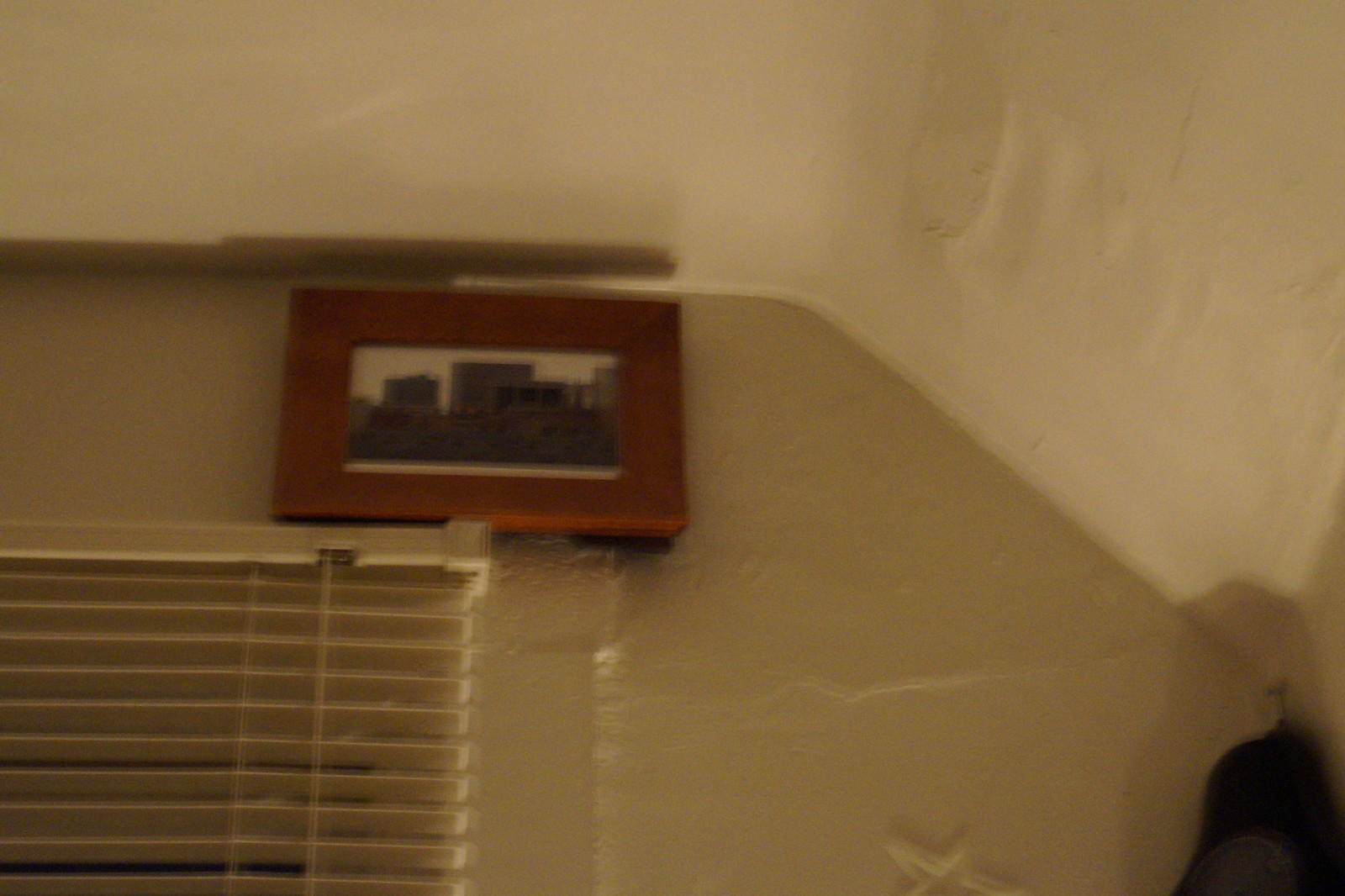The image depicts a blurry photograph of a room's upper area, focusing on the intersection of the ceiling and walls. The ceiling and walls are painted an off-white hue, with noticeable texture, and some sections appear slightly yellowed due to potential water damage. The ceiling lacks crown molding and shows a curved slope downwards to the right, suggesting it might be the top floor of the house. Towards the top left, there are brown streaks, likely indicating incomplete paintwork. 

A wooden picture frame hangs directly below the ceiling, nearly touching it. The frame encases an indistinct image, possibly of a cityscape or buildings, depicted in gray tones against a white backdrop. Positioned above a window with closed, traditional white blinds on the bottom left, the room seems to be captured at night, inferred from the darkness visible through the blinds' cracks. In the bottom right corner, part of a black object, possibly a hook or hanging item, is visible, adding a subtle detail to the otherwise plain setting.